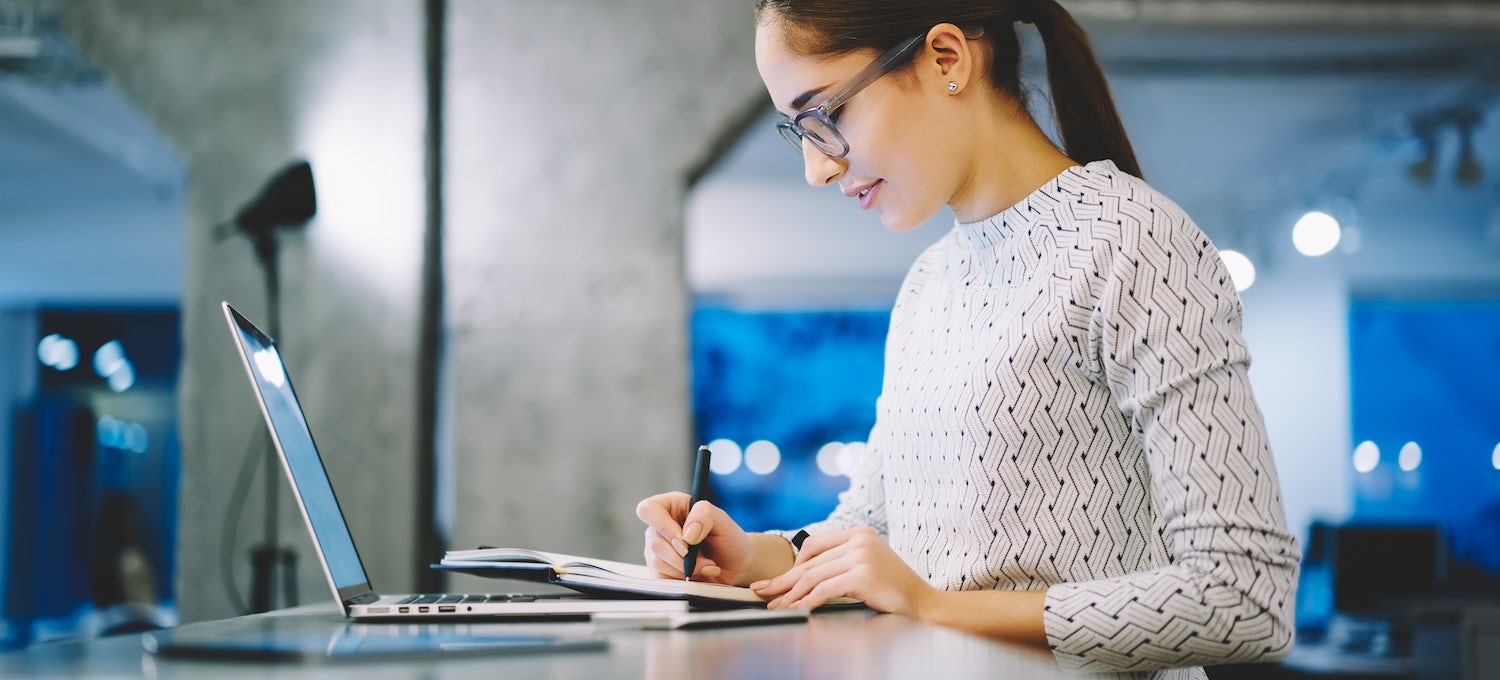The photograph captures a high-quality, professional profile view of a young woman engrossed in her work, suitable for a website or similar professional use. She is wearing a white, geometric-patterned top, complemented by diamond stud earrings and smoky gray eyeglasses. Her long brown hair is neatly pulled back into a ponytail. The woman is writing in a black book or planner with a small stubby black pen, while an open, slim laptop sits on the desk in front of her. The setting is a modern open office space, with multiple workspaces visible behind her, though they are out of focus. A gray concrete pillar, illuminated by an external light source, stands out in the background. The scene captures her dedication as she looks down at her work, her attention fully absorbed by the task at hand.